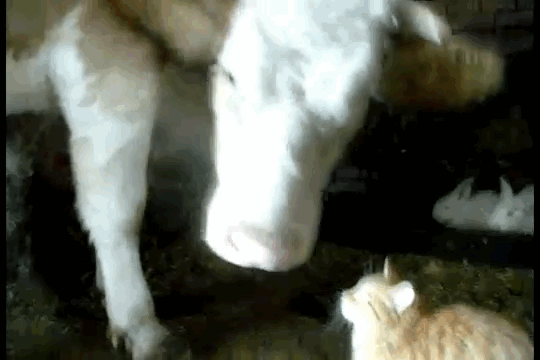In a cozy barn setting, a white cow with brown ears and gray hooves is seen in the upper left-hand corner of the image, standing against a backdrop of hay-strewn floor. Dominating the scene, the cow is tenderly nudging an orange cat located in the bottom right-hand corner, then proceeds to lovingly lick the cat’s head and back down towards its tail. Adding to the charming farm tableau, a black tray with two white bunnies, seemingly engaged in a meal, is visible in the background. This heartwarming image captures a moment of interspecies affection amidst a rustic barn environment.